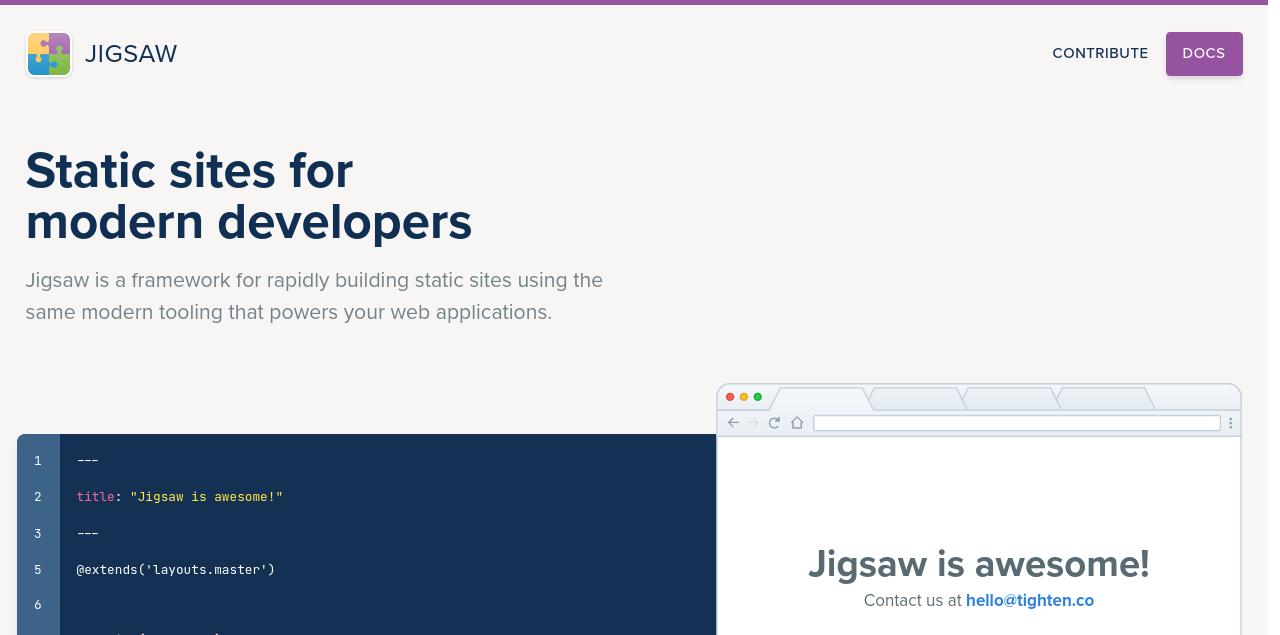This website screenshot features a thin purple border lining the top edge. In the top left corner, the name "JIGSAW" is prominently displayed in uppercase letters, immediately adjacent to a logo consisting of four interlocking puzzle pieces colored yellow, purple, green, and blue, arranged in a clockwise manner. Below this, the headline "Static Sites for Modern Developers" is presented in large, bold blue letters. A subheadline in smaller, gray text reads, "Jigsaw is a framework for rapidly building static sites using the same modern tooling that powers your website applications."

Beneath this, there is an image of a code snippet in a blue box, displaying the text:
```
title: Jigsaw is awesome
@extends layout.master
```
To the right of the code snippet, there is a partial browser window screenshot. The current tab in the browser reads "Jigsaw is awesome!" and multiple other tabs are visible. Below the browser, the text "Contact us at hello@titan.co" is shown, with "Contact us at" in gray and the email address in blue.

In the top right corner of the website, there are two buttons: one purple button labeled "Docs" and another labeled "Contribute."